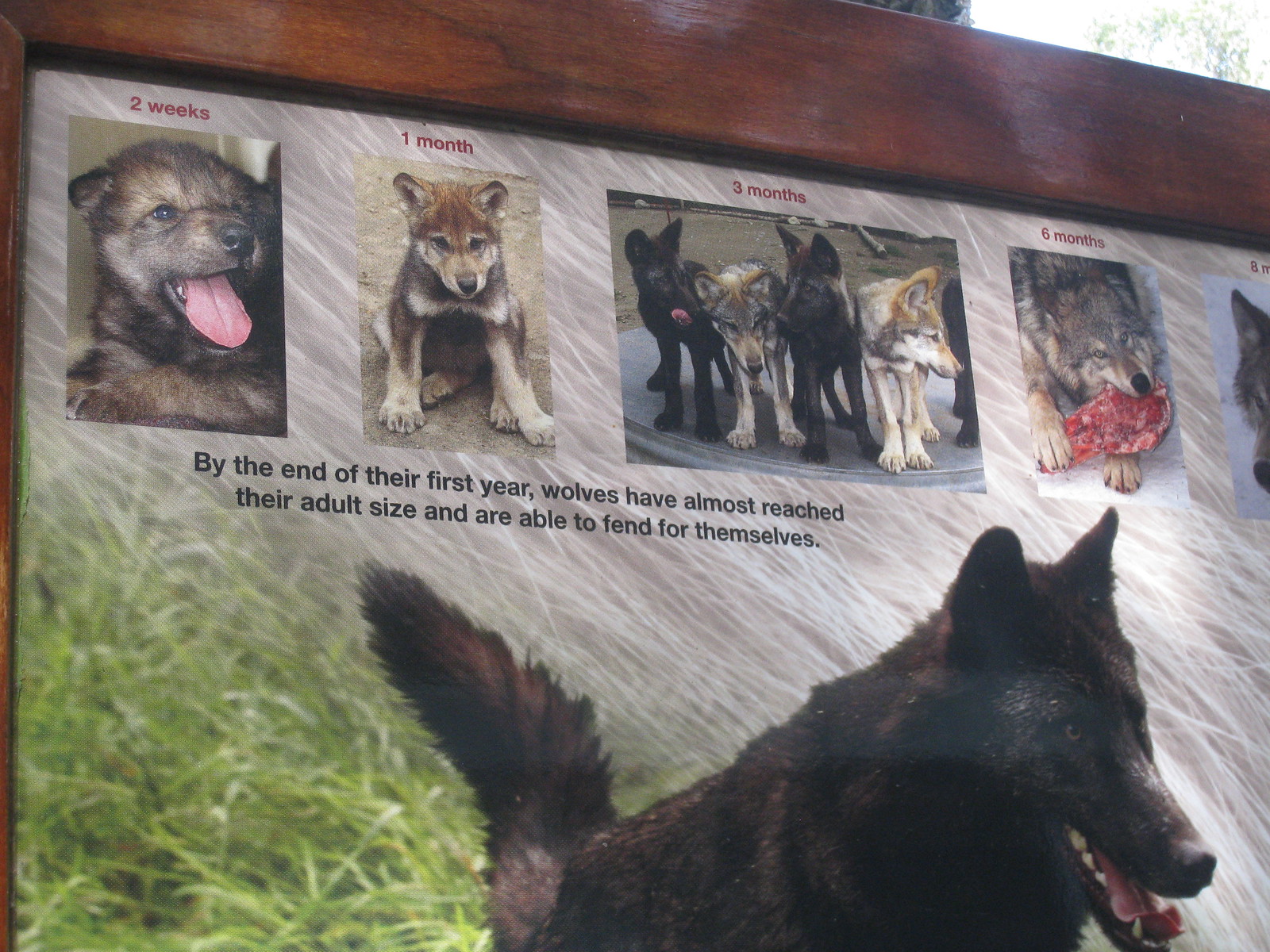The image is a wide, rectangular photograph that appears to be part of an educational sign, possibly located in a wild park or forest, depicting the growth stages of wolves. The photograph is framed in thick, dark brown wood, which can be seen sloping diagonally from the top of the image and partly on the left side. In the background, a green grassy area covered in white hay is visible. At the bottom right corner, there is a large, dark brown wolf resembling a dog, facing the right edge of the frame.

Above this wolf, the sign features a timeline with small images of wolves at different ages, accompanied by red text. It starts with a wolf pup at "two weeks," then shows another at "one month" resembling the size of a Shiba Inu, followed by a "three months" image where the wolf is the size of a Golden Retriever. At "six months," the wolf appears almost fully grown, depicted as slightly terrifying with a raw piece of meat in its mouth. There is also an image at "eight months," although details about this image are unclear.

Below each image, black text reads: "By the end of their first year, wolves have almost reached their adult size and are able to fend for themselves." This educational message underlines the rapid growth and development of wolves within their first year.